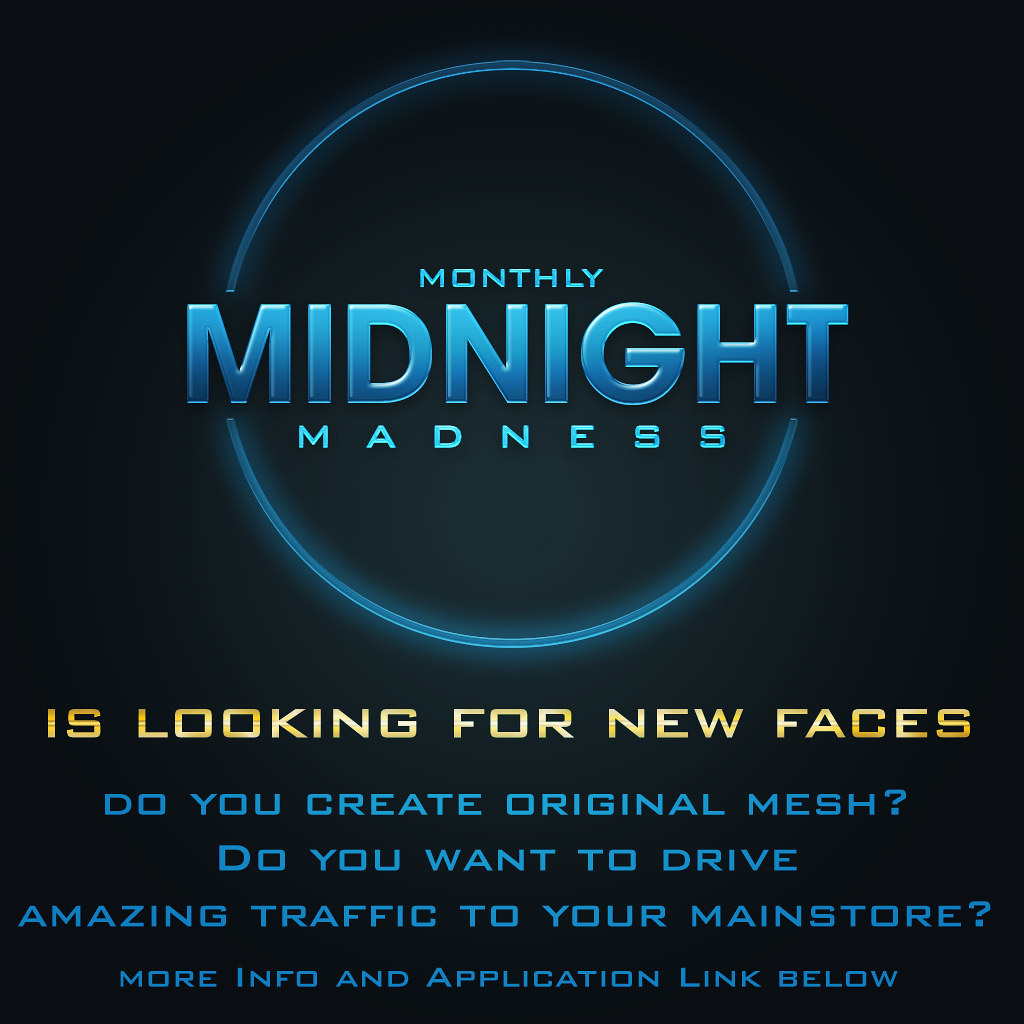This digital event flyer is predominantly black with a sleek, modern design intended for social media platforms such as Facebook or Instagram. The upper half of the image features a glowing light blue circle containing the text "Monthly Midnight Madness," with "Midnight" prominently displayed in a larger, beveled glass font, giving it a 3D effect. The words "Monthly" and "Madness" are smaller and lighter in color. Below this captivating logo, the text in gold letters reads, "Is looking for new faces." Further down, the flyer includes additional information: "Do you create original mesh? Do you want to drive amazing traffic to your main store? More info and application link below." The overall design is visually striking, with the contrast between the light blue, gold, and black elements capturing attention effectively.